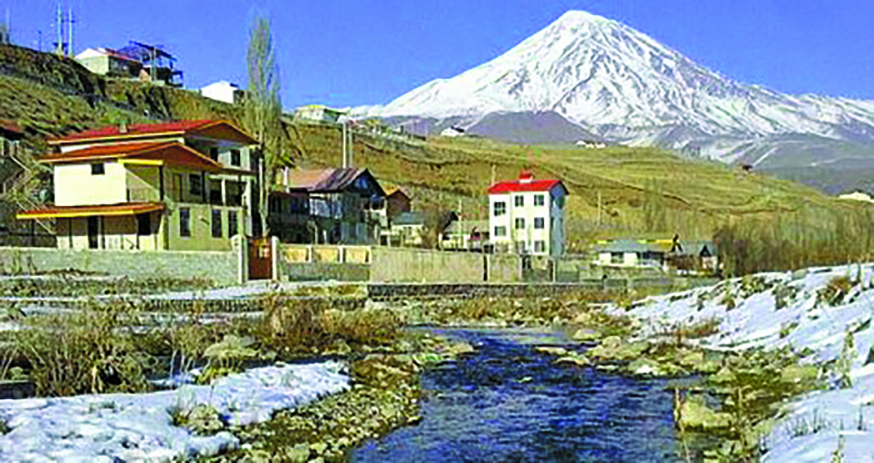In this grainy photograph, a serene and snowy winter landscape unfolds, dominated by a towering, snow-covered mountain range in the background. The scene is set in a small, rural settlement nestled at the foot of the mountain. The snow blankets the ground and hill areas on both the right and left sides of a calm, narrow river that flows straight down the middle of the image, flanked by shrubs and melting snow, indicative of an early thaw.

In the village, a variety of buildings are scattered across the landscape, built across different elevation levels, contributing to the scene's picturesque quality. The settlement features modern structures, likely from the 1990s or 2000s, with distinctive roofs—orange, red, and grey—standing out against the wintry setting. Especially notable is a tall, narrow building with a red roof in the center, accompanied by other lower buildings with various colored roofs, including a green one. These structures are enclosed by a cement wall, adding a touch of structure to the otherwise desolate scene.

A road runs along the settlement and beside the river, but no signs of human presence can be found, reinforcing the tranquil and peaceful atmosphere of this rural town. The absence of people and trees, along with the short grass on the hills, accentuates the stillness, making it a perfect snapshot of a quiet, snow-covered winter day.